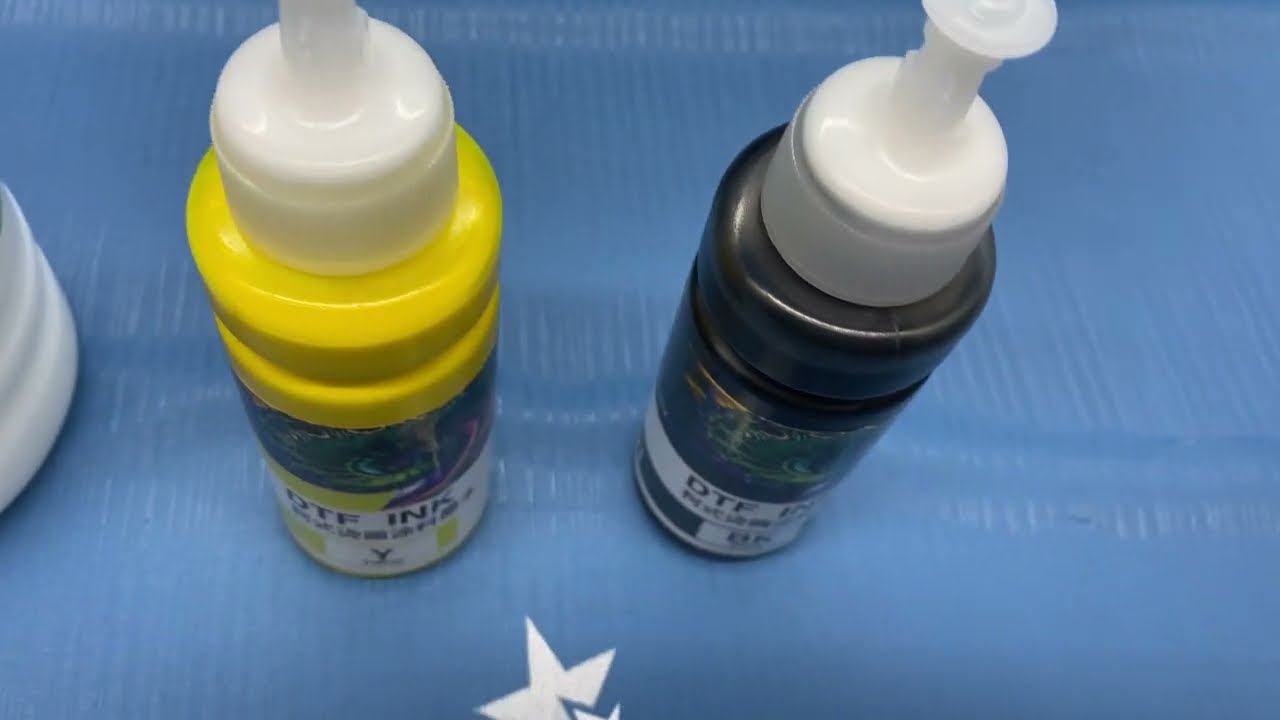The photograph captures a close-up of a blue table covered with a fabric tablecloth, displaying subtle parallel stripes. At the bottom edge of the image, slightly off-center, is a white star symbol, with only three points of a larger star and an outline of a smaller one visible. The centerpiece of the image consists of two bottles of paint positioned next to each other. The bottle on the left contains yellow paint and features a white cap along with a black-and-white label that reads "DTF INK." This label includes some green and light blue swirly patterns. The bottle on the right contains black paint, also with a white cap and a similar label that reads "DTF INK." A faint additional mark, potentially another letter or number, is visible but partially faded. Adjacent to these paint bottles is an additional white object, whose details are not clearly described.